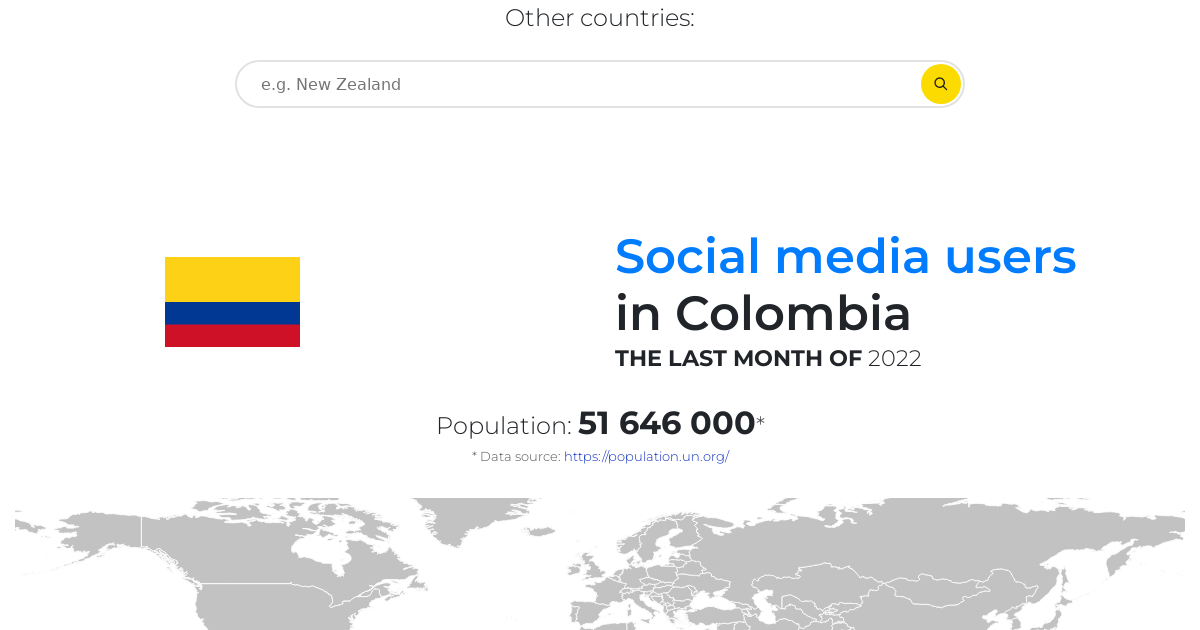A detailed and cleaned-up caption for the described image:

"The image prominently features a composite map display divided into two sections. At the top, there is a search bar indicating 'New Zealand' alongside an option for social media users highlighted in blue. Beside these elements, details about Colombia are presented, including its population of 51,646,000 as of the last month of 2022, sourced from populationun.org. Adding to this information, the Colombian flag is displayed on the left side, characterized by a large yellow stripe atop thinner blue and red stripes.

Below, a black and white map showcases the majority of North America, including the lower half of Greenland, Iceland, Canada, and Alaska. Extending across the Atlantic Ocean, the map also features the entirety of the European Union, parts of Russia, China, including the left part of the Gobi Desert and eastern regions, as well as Japan and Kazakhstan. This detailed representation seems to depict a global social media search platform, providing country-specific data and geographical context."